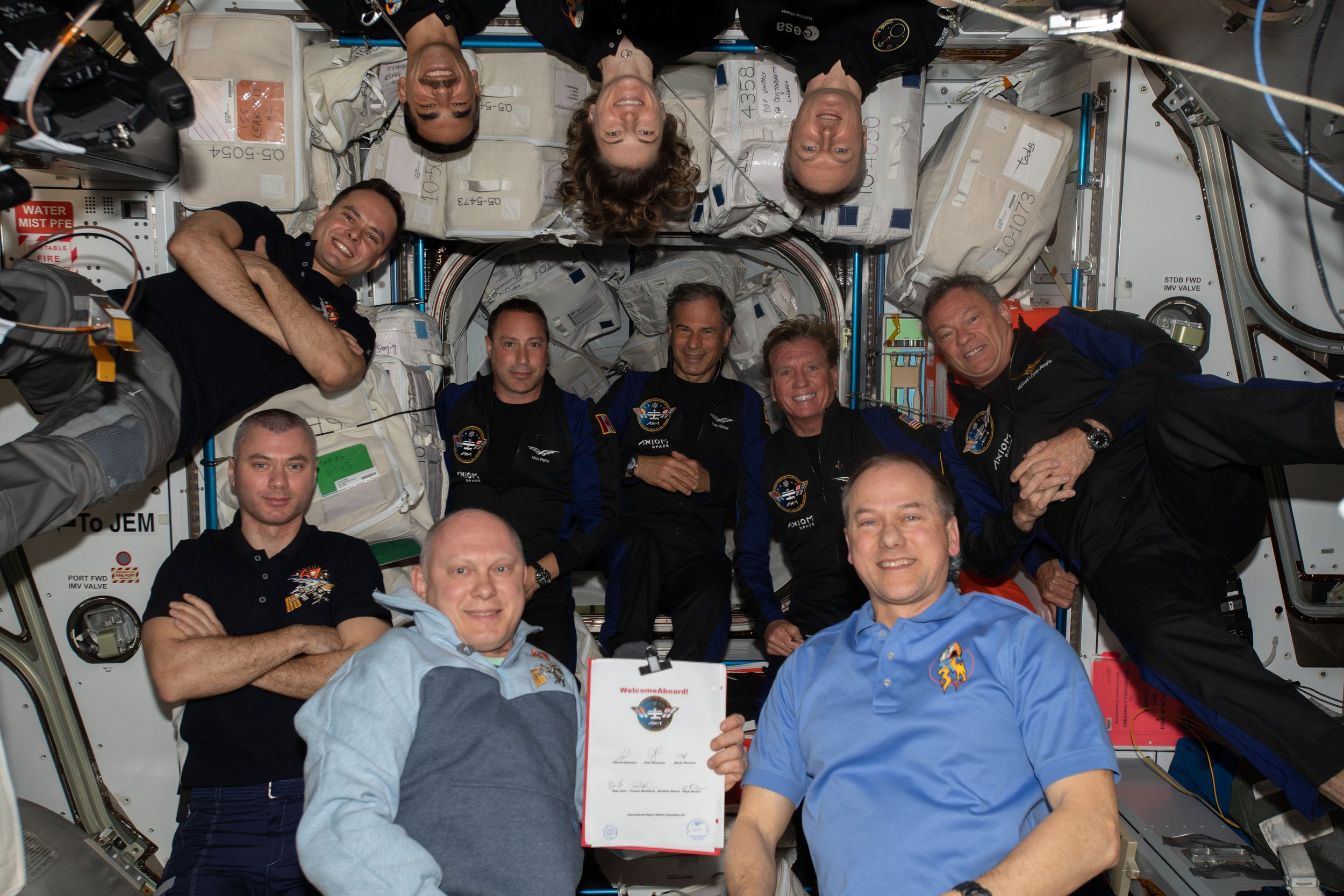This full-color photograph taken inside the International Space Station captures a busy scene of eleven astronauts, highlighting the camaraderie and weightlessness of the environment. In the foreground, two white men are prominently positioned; the man on the left wears a light blue and gray shirt, while the man on the right sports a light blue collared shirt. They are holding up a clipboard with space documents, projecting a sense of professionalism and focus. Surrounding them are their crewmates, who are dressed in dark-colored uniforms adorned with space program logos on the right breast. The backdrop features a total of eleven astronauts, consisting of mostly men and a notable inclusion of three women, who are distinguishable by their orientation—three faces hanging upside down from the top of the frame, adding a unique, humorous touch to the photograph. The arrangement and expressions—most of them smiling—capture a moment of unity among the crew. The walls of the station are lined with compartments and packages, secured with straps, providing insight into the organized living and working space. Overall, this image vividly illustrates the dynamic and collaborative nature of life aboard the International Space Station.